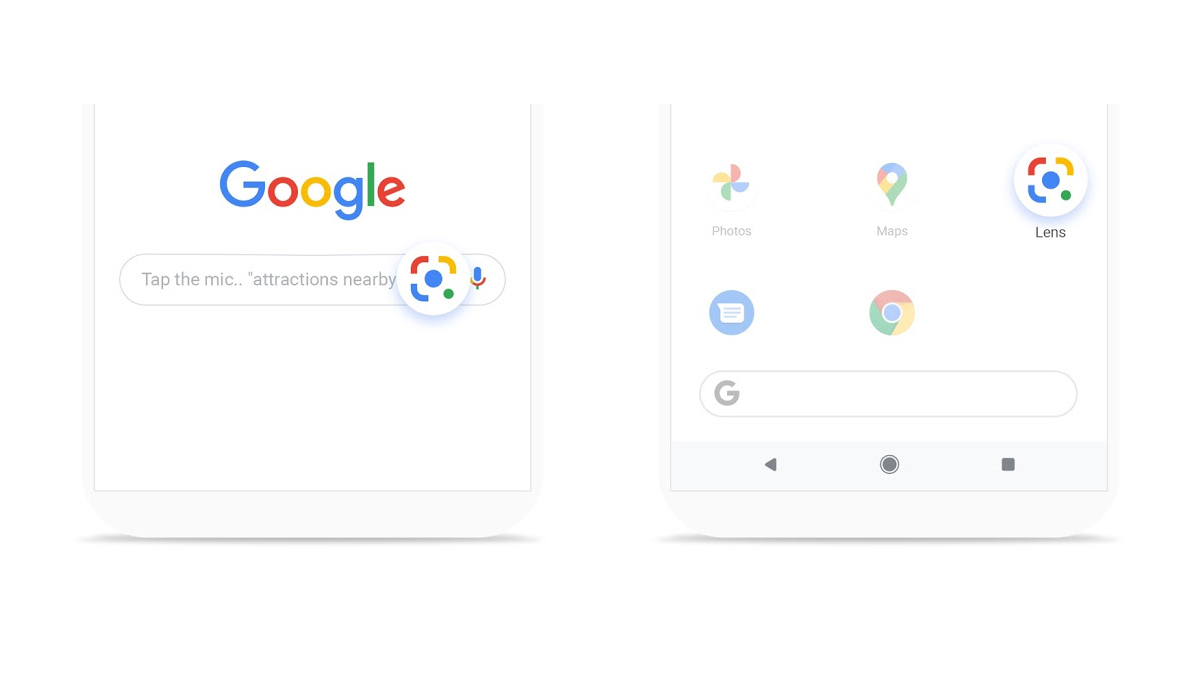The image consists of two tiled screenshots side-by-side. On the left is a screenshot of a mobile Google search page. The page prominently displays the large, colorful Google logo at the top with a text input box beneath it. Within the input box, there is a Google Lens button, marked by an elbow-noodle-shaped outline in red, yellow, and blue with a small dot in the lower right-hand corner and a larger dot in the middle, symbolizing a camera function. Adjacent to the Google Lens button is a blue and red microphone icon. The search box text prompt reads "Tap the mic, attractions nearby."

The right-hand screenshot features a Google menu. At the top, there are visible options such as Photos and a blue Pinwheel icon, followed by a Maps button. The Lens icon is selected, indicating that the Google Lens feature is active. Below the Lens icon, there appears to be a Messages button characterized by a classic blue text box icon, and a Chrome logo which consists of an outer ring made up of segments in red, yellow, and green, with a blue dot in the center. The bottom of the screen shows standard phone navigation buttons: a back button on the left, a home button in the center, and a square on the right for multitasking or going forward.

Overall, the image provides a detailed view of the user interface elements and icons on a mobile Google search page and a Google menu, demonstrating various functionalities available on a smartphone.